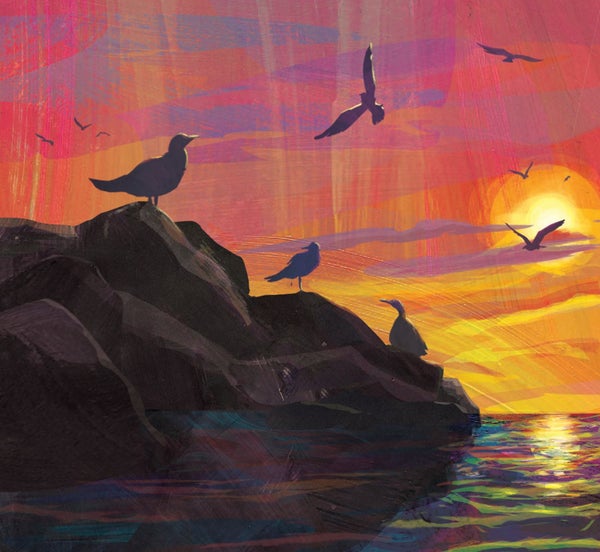The painting depicts an impressionistic ocean scene during a vibrant sunset, rendered in what appears to be either watercolor or oil paint, characterized by its delicate interplay of colors and textures. The sky is an arresting tapestry of bright oranges, reds, purples, and hues of blue, seamlessly blending into a mesmerizing dusk. On the horizon, a yellow sun, partly veiled, casts its radiant glow across the scene, creating vivid reflections in the water below.

In the serene foreground, a jagged, dark gray rock formation rises from the multicolored water - a dynamic mix of purple, green, blue, and yellow thanks to the sun’s reflection. Perched upon this rocky outcrop are three silhouetted seagulls: one at the pinnacle on the left, another positioned centrally slightly lower, and the third at the bottom right.

In the sky above, a collection of birds, totaling eight, is captured in mid-flight. Their silhouettes punctuate the ethereal backdrop; three smaller birds to the left, another trio to the right, while a larger bird with outstretched wings dominates the central sky alongside a smaller companion with wings held upward toward the sun. This masterful blend of natural elements and avian life exudes tranquility and captures the sublime beauty of nature at dusk.